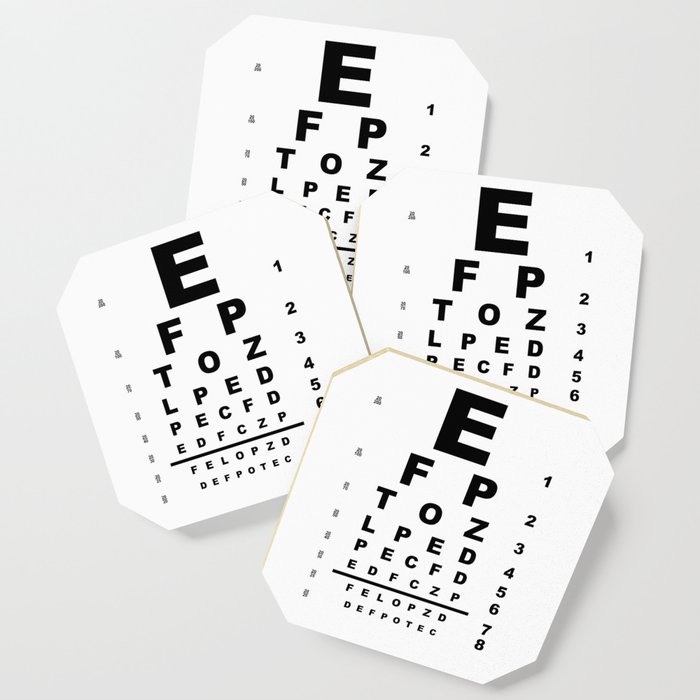The image features four identical eye charts, commonly used for vision testing, arranged on a pure white background in a slightly overlapping manner. The charts are layered: one in the back, two in the middle overlapping each other with the left one slightly covering the right, and the fourth in the front overlapping the middle two. Each chart begins with a large, bold letter 'E' at the top, followed by progressively smaller letters as you move down. The sequence of letters reads: 'E' on the first line, 'F P' on the second, 'T O Z' on the third, 'L P E D' on the fourth, 'P E C F D' on the fifth, 'E D F C Z P' on the sixth, 'F E L O P Z D' on the seventh, and 'D E F P O T E C' on the eighth. Though the charts appear to be lying flat, shadows suggest a top-down view. Additionally, there are small symbols to the left of each row, but they are too small to discern in this resolution.